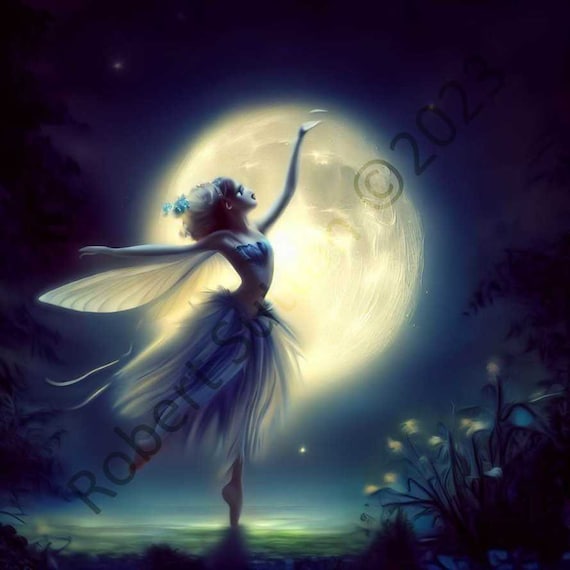This digitally created illustration captures an ethereal fairy standing gracefully on her tiptoes in a ballerina pose against a dark night sky, highlighted by a large, glowing moon. The fairy, adorned with delicate, feather-like wings and a feathery tutu, exudes an airy and light presence. Her form-fitting top and wisp-thin figure contribute to her otherworldly elegance. A blue ribbon adorns her hair as she holds her hand up towards the sky. Yellow glowing flowers at her feet add a magical touch to the scene, complementing the moon's soft light. The lower right corner features a barely readable copyright watermark by Robert S. Yu, marking this enchanting artwork.